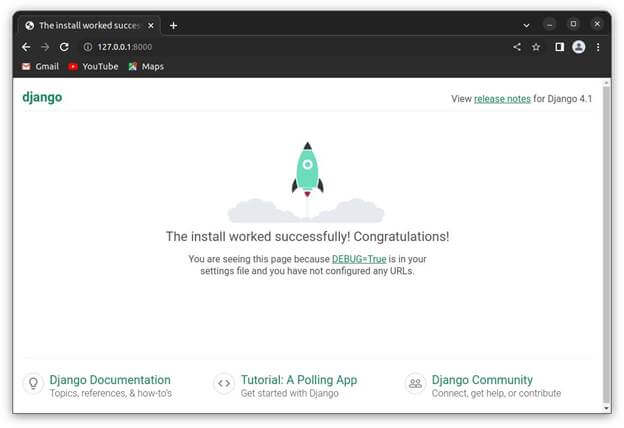The image showcases a Django website interface. At the top left, the word "Django" is prominently displayed in green text. Dominating the center is an illustration of a rocket ship, which is light green with a white circle in its middle, ascending vertically. Beneath the rocket, the message "The install worked successfully. Congratulations!" is displayed, followed by a note stating, "You are seeing this page because 'DEBUG=True' is in your settings file and you have not configured any URLs." The term "DEBUG=True" is highlighted in green text. 

In the top right corner, there's a link to "View release notes for Django 4.1," with "release notes" also in green text. The bottom section of the image is divided into three distinct areas. On the bottom left, "Django documentation" is displayed next to a small circle containing a bell icon. The bottom center features the text "Tutorial: A Polling App," accompanied by a circle on its left that has arrows pointing left and right. Finally, on the bottom right, "The Django community" is shown next to a circle containing icons of two people.